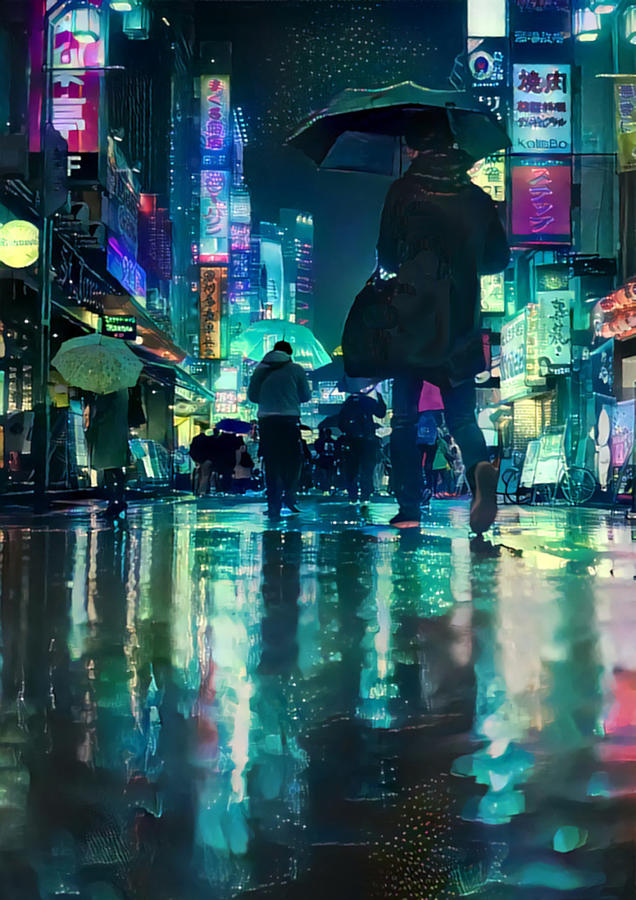The image depicts a vibrant and colorful night scene of a modern city street, likely in Tokyo, characterized by its bright, illuminated billboards and neon signs adorned with Asian characters. The scene is set on a rainy night, as evidenced by the reflections and puddles on the wet pavement. Numerous people, clad in coats and hoods, walk along the street under an array of vividly colored umbrellas, with some individuals walking towards the camera and others away from it. The street is bustling with life, featuring details such as a bicycle, various signs, and storefronts along the roadside. The dominant hues of pink, purple, green, and blue add to the overall lively and dynamic atmosphere of the cityscape.